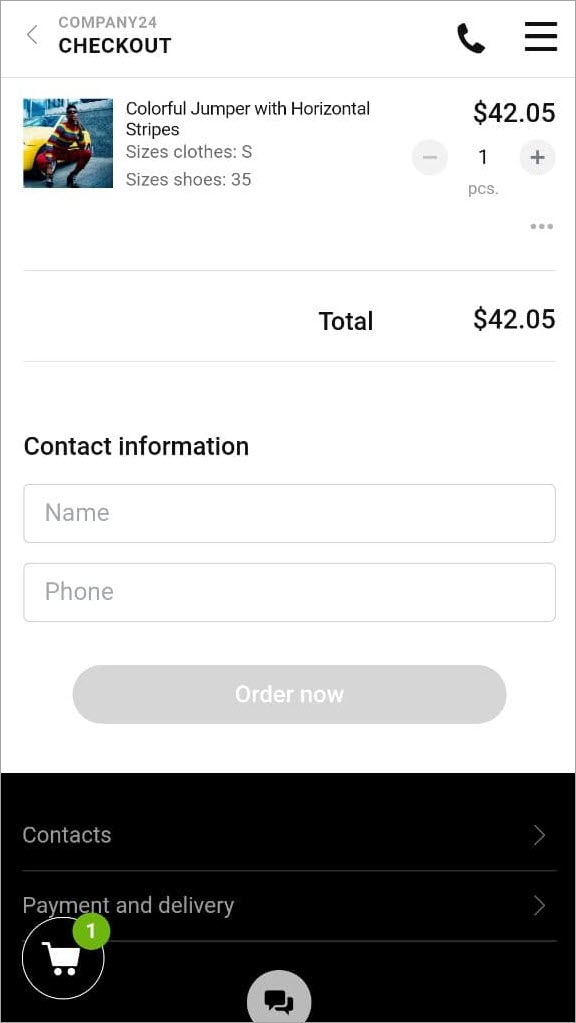Here is a detailed and refined caption for the image:

---

The screenshot displays a smartphone interface with a sleek design. At the top, a light gray bezel bears the text "Company 24" and "Checkout" in bold black. On the top left, a light gray arrow is visible, while on the top right, there is a symbol of a phone, followed by three bold black lines representing a menu.

Below the bezel, a new section showcases an individual crouching in front of a yellow car. The person is dressed in red pants and a distinctive long-sleeved shirt featuring horizontal stripes in red, yellow, and green. To the right of this image, the text "Colorful Jumper with horizontal stripes" appears, with the price "$42.05" in bold black directly below it.

Further down, the interface provides size options. Sizes for the "Jumper" are listed with "Close... S for small," accompanied by a gray circle containing a darker gray minus sign, a number "1" in black (indicating one piece), and another gray circle with a darker gray plus sign for adjusting the quantity.

To the left, sizes for shoes are noted as "35" in gray. At the bottom of this section, the total cost is reaffirmed as "$42.05."

The "Contact Information" heading is in black, followed by two gray-bordered rectangles labeled "Name" and "Phone" for user input. Centrally positioned at the bottom is a dark gray button with "Order Now" inscribed in white.

In the black footer section, gray text along with gray arrows point to "Contacts" and "Payment and Delivery" options. Additionally, a black circle encloses a green circle with a white "1," adjacent to a white shopping cart icon. A gray circle at the bottom contains two black chat bubbles facing opposite directions.

---

This caption provides a comprehensive description of the image, highlighting all the key elements and their respective positions in the user interface.